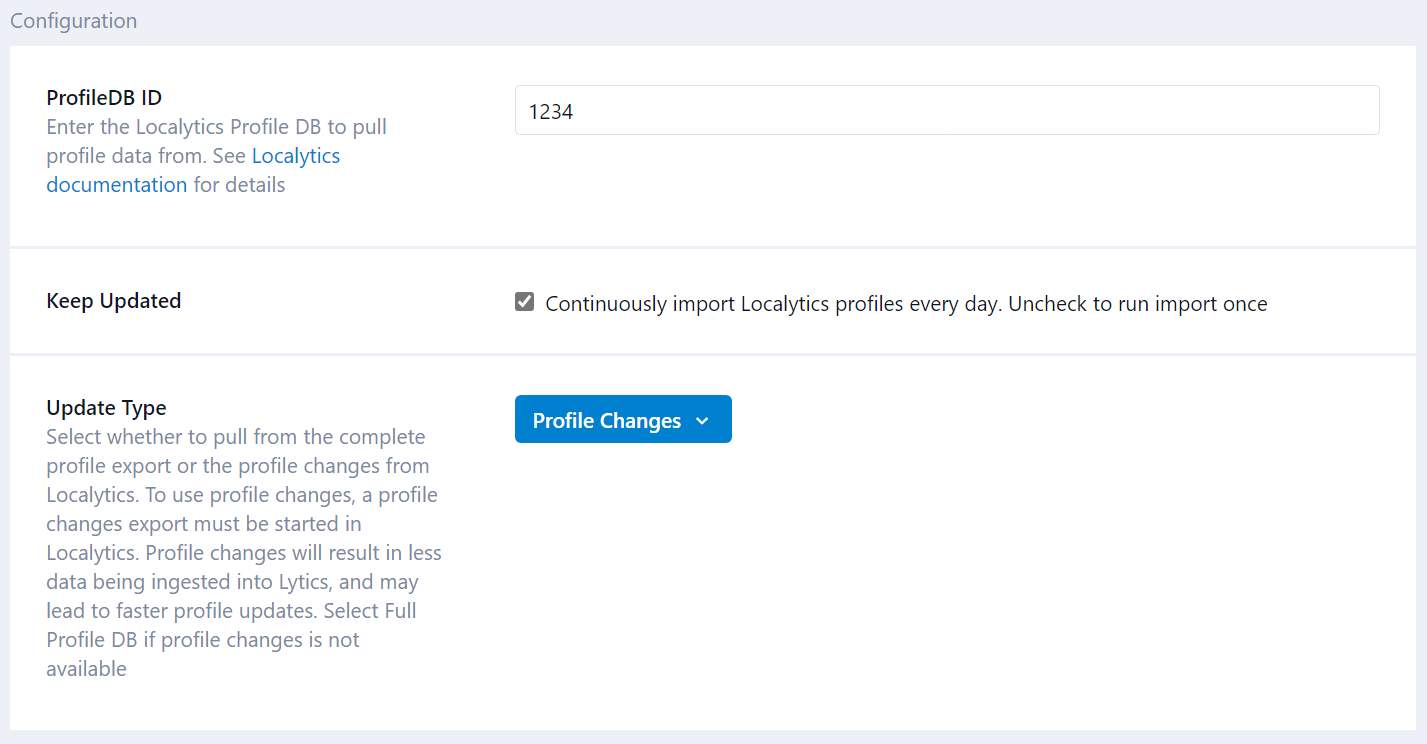This image is a screenshot from a utility page with a clean, white background. At the very top, there is a very light gray border with a bluish tint. 

In the upper left corner, the word "Configuration" is written in gray font. Directly below, in black font, it says "ProfileDB," with "DB" capitalized and attached without a space to "Profile." 

Next, there's a field labeled "ID," followed by a gray font instruction: "Enter the Localytics Profile DB to pull profile data from." Beneath this, in blue font, is a hyperlink text: "See Localytics documentation for details."

On the right side of the page, there is a long, outlined rectangle in very light gray suggesting an input field. Inside this field, it displays "1234."

Further down, there is a section labeled "Keep Updated." To its right, the text reads: "Continuously import Localytics profiles every day. Uncheck to run import once." The checkbox adjacent to this text is marked, indicating the daily import preference.

At the bottom, there’s a category named "Update Types," accompanied by a lengthy detailed description, all in gray font. To the right, there's a blue rectangle button with white text that reads "Profile Changes," and a downward-pointing white arrow to the right, suggesting a drop-down menu.